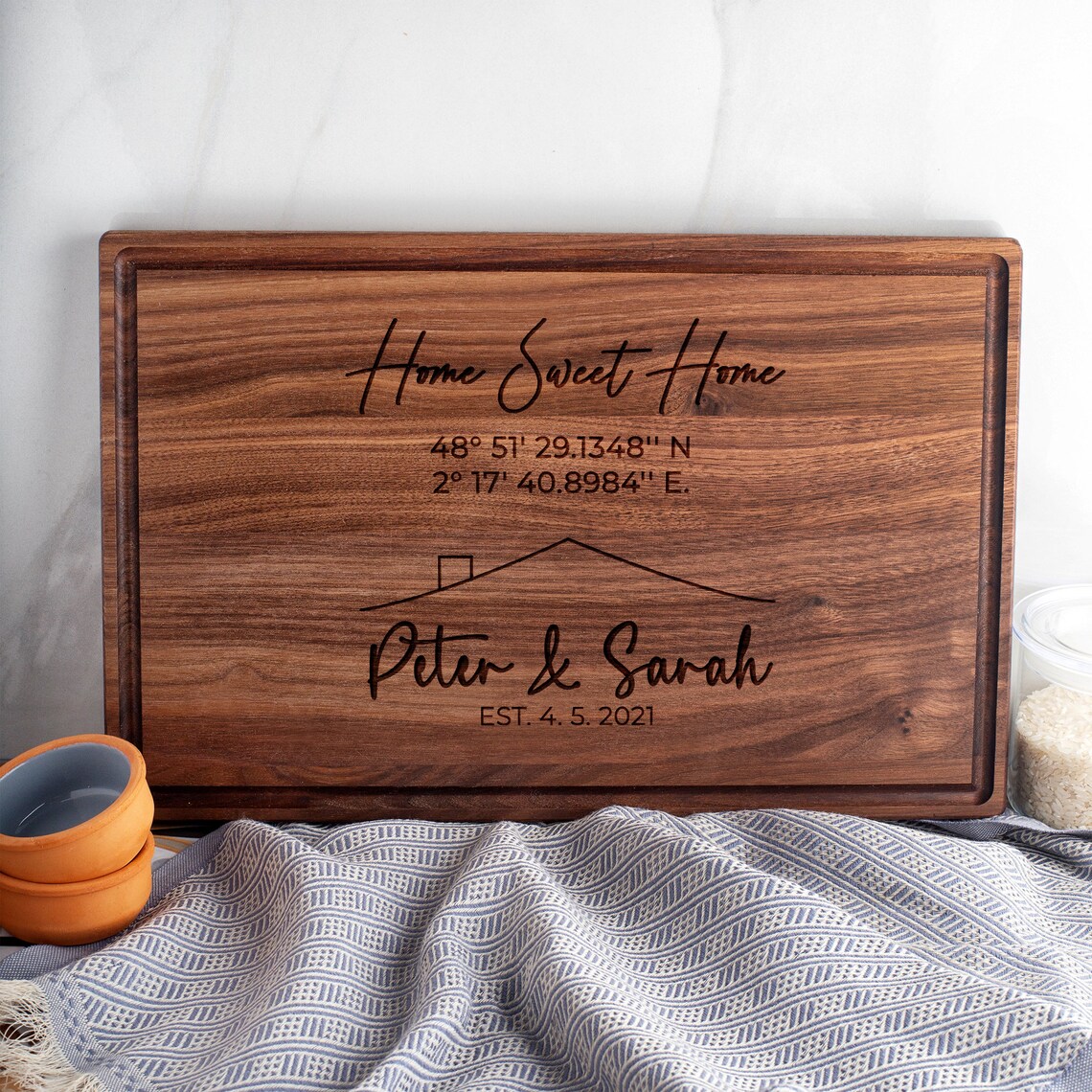The image features a detailed wooden plaque, precisely crafted and leaning against a white wall with a marbling effect. The plaque is positioned atop a blue and white checkered linen with frilled edges, which seems to be a blanket. To the left of the plaque are two small orange bowls, each with a blue interior, while on the right, there is a clear tub containing what appears to be grains of rice. This rectangular wooden plaque, finished with a natural brown varnish, features an engraved border that adds depth and a polished feel. The plaque prominently displays "Home Sweet Home" at the top in cursive lettering, followed by specific geographical coordinates: 48 degrees 51' 29.1348" N, 2 degrees 17' 40.8984" E. Below the coordinates is a detailed etched illustration of a house roof with a chimney. Further down, in elegant script, it reads "Peter and Sarah EST 4.5.2021."